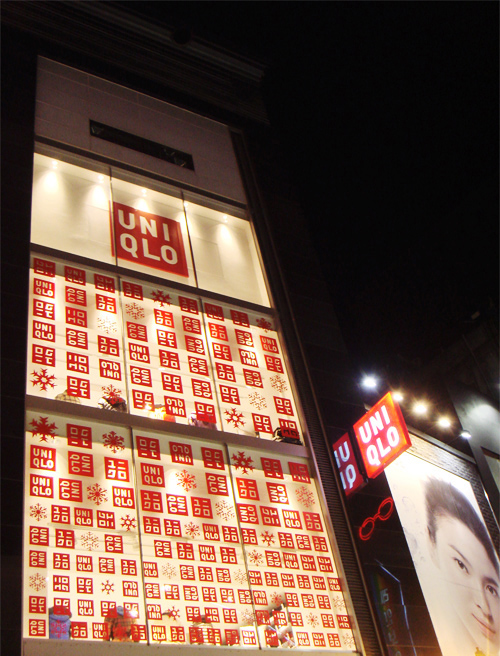The photograph, taken at night, captures an urban scene likely in a bustling Asian city such as Tokyo or Hong Kong. The sky is completely black, devoid of stars, highlighting the prominence of the illuminated structures and advertisements. Central to the image is a large rectangular display on the side of a towering building. This display features bright white sections interspersed with red blocks containing text and symbols, possibly in an Asian language. Dominating the top of the display is a prominent red square with the text "UNI QLO" in capital letters. Below this, a grid of persistent red squares continues downwards, forming a dynamic pattern.

To the right of this primary display, another large sign protrudes from the building, also featuring the "UNI QLO" branding. Above this secondary sign, a series of stage lights shine down, adding to the overall brightness of the scene. There's a black and white photograph of a person—gender ambiguous—looking towards the camera, further enhancing the urban vibe. Additionally, to the right of this photo, a smaller, well-lit advertisement includes a pair of red eyeglasses. The well-lit buildings starkly contrast the pitch-black sky, making the vibrant signage and illuminated ads stand out in the nocturnal cityscape.